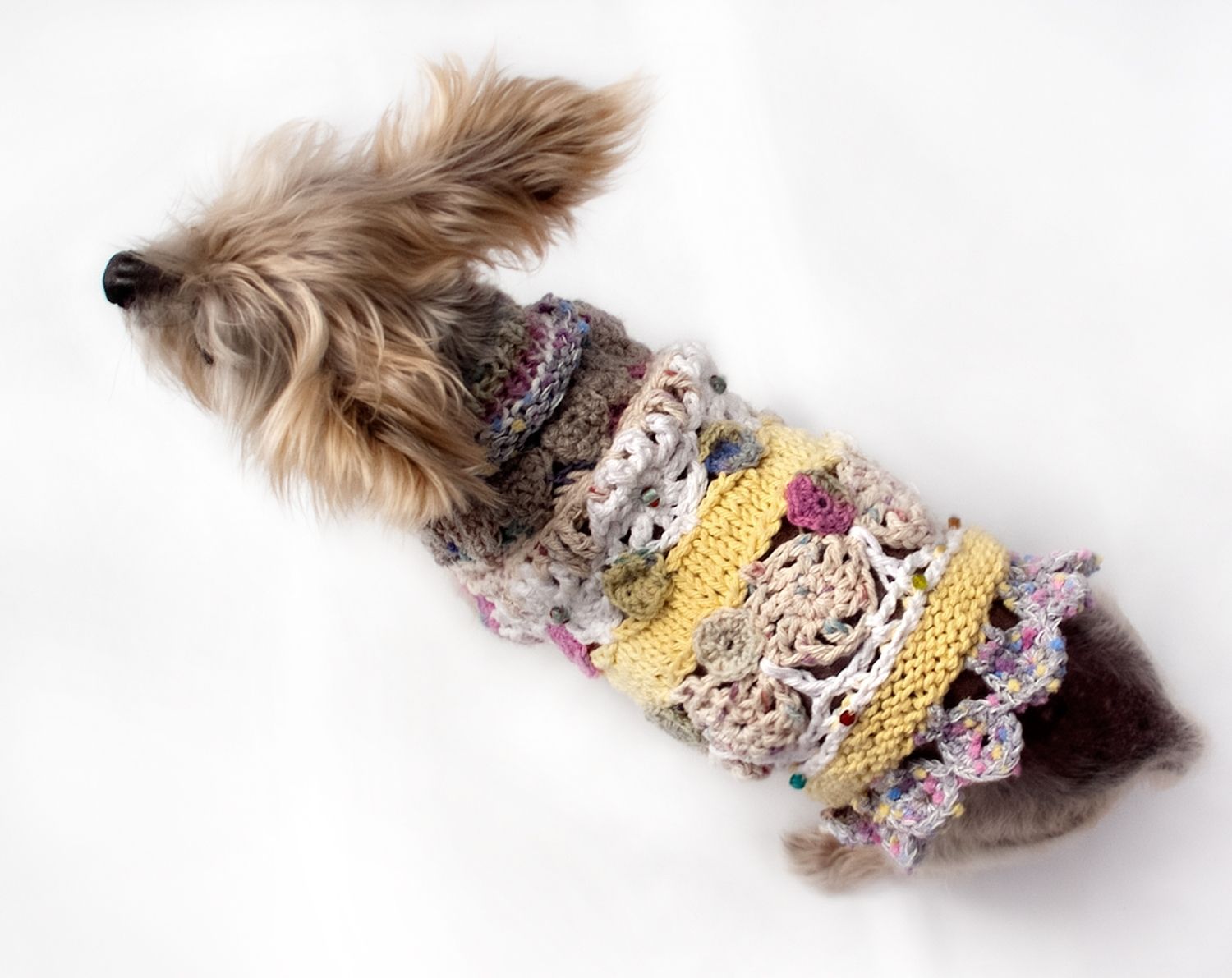The photograph showcases a cute Yorkie, positioned with its back near the bottom right and its nose pointing towards the top left corner, against a pure white background. The Yorkie's fur is a striking combination of golden on its head and feet and silvery-grey across its body. The little dog is adorned in a homemade, pastel, knitted sweater that extends from its neck to the bottom of its waist, decorated with delicate hearts, flowers, and yellow yarn bands. The image captures the Yorkie from above, giving a clear view of its charming attire, and it looks as if the dog’s attention is drawn off-camera, conveying a sense of engagement that suggests a photo shoot to highlight the adorable sweater.